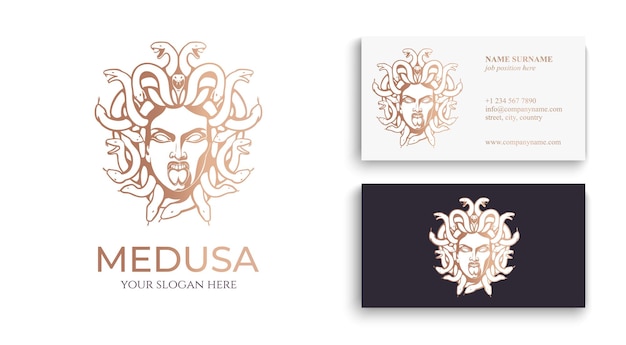The image showcases a detailed template for a business card printer named Medusa. On the left side, there is the Medusa logo, featuring an ominous image of an angry woman with a forked tongue, monochromatic eyes, and snakes writhing around her head, each facing different directions. The logo is outlined in tan and is accompanied by the text "Medusa" in brown, followed by "your slogan here" in black underneath. To the right, two business cards are displayed. The top card has a pristine white background with the Medusa logo on the left and a layout on the right for personal and business information including name, surname, job position, phone number, email, street, city, country, and website. Below it is the reverse side of the card, featuring a stark navy blue or black background with the Medusa logo prominently centered.